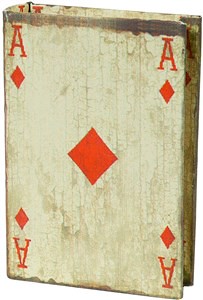Upon first glance, the image appears to depict the Ace of Diamonds card, recognizable to those familiar with card games. Characteristically, the Ace of Diamonds is marked by a single, centrally located red diamond and features a capital 'A' in the top corners: left and right, as well as the bottom corners: left and right. However, a closer examination reveals that this image may actually show a carrying case designed for a deck of cards. This conclusion arises from the noticeable spacing between the apparent front panel and the back panel, as well as the presence of discernible third and fourth sides. Specifically, the top left-hand side suggests a connection between the front and back, indicative of a hinged or bound structure. Meanwhile, the ambiguity of the closure on the right-hand side leaves some uncertainty. This could alternatively suggest that the object is a book cover, possibly of a durable or hardcover nature, due to the visible structural elements on both the top and sides.